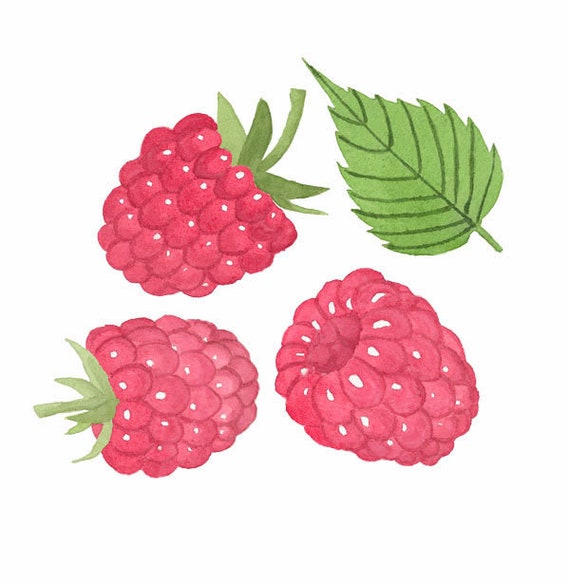The image is a highly detailed and vibrant color illustration depicting three raspberries and a leaf, arranged in a loose square formation. Each raspberry is illustrated from a different angle, showcasing the fruit's rich, deep reddish-pink hues and the intricate white highlights that give depth to the seeds. The top raspberry is positioned with its stem attached, pointing downward to the left. Below it on the left, another raspberry is shown from the opposite angle, pointing down to the right with its stem also intact. To the right of this, there is a raspberry missing its leafy stem, revealing the cavity where the stem used to be. Above this bottom-right raspberry, a lush green leaf is intricately drawn, appearing freshly plucked from the fruit. The illustration is rendered in a pastel style, giving it a soft, cutesy vibe, yet it displays the artist's talent through the accurate and vibrant representation. The background is a clean white, making the colors pop, reminiscent of illustrations one might find in a detailed guide to different kinds of fruits.